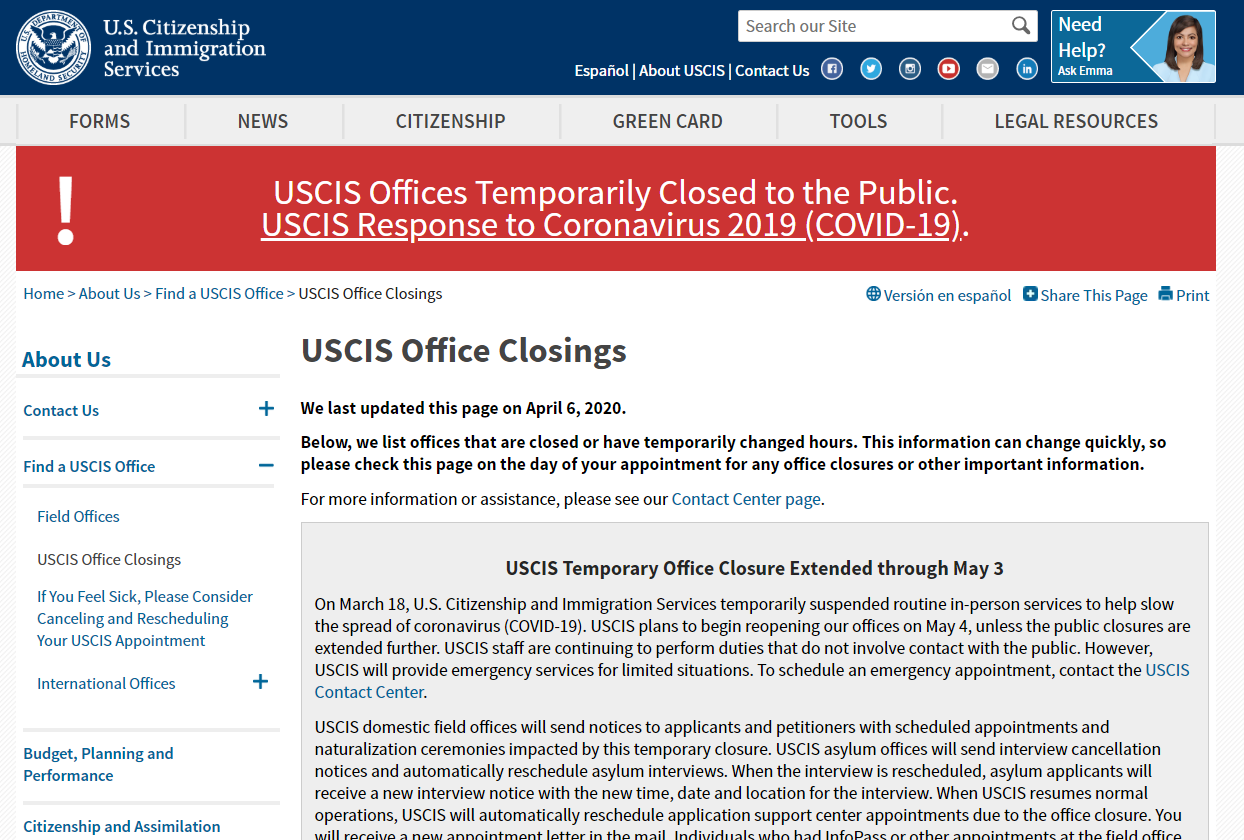Here’s a cleaned-up and detailed caption for the described image:

---

The screenshot depicts a web page from the U.S. Citizenship and Immigration Services (USCIS) website. At the top, there is a prominent horizontal blue border. On the left side inside the blue border, the USCIS name is displayed alongside a circular logo featuring an eagle and accompanying text. On the right side of the blue border, there is a search box with options underneath it that read "Español," "About USCIS," and "Contact Us." Adjacent to these options are social media icons. The far-right corner of the border features a rectangular graphic with a headshot of a woman and the text "Need Help? Ask Emma."

Below the blue border is a horizontal gray navigation menu with black text. The menu includes sections labeled "Forms," "News," "Citizenship," "Green Card," "Tools," and "Legal Resources." 

Directly beneath the gray menu is a bold red emergency notification bar that stretches across the page. On the left of the bar, there is a white exclamation mark, and the main message reads: "USCIS Offices Temporarily Closed to the Public. USCIS Response to Coronavirus 2019 (COVID-19)."

Following the emergency notice, there is an article titled "USCIS Office Closings," which states in small letters that the page was last updated on April 6, 2020. The article provides details about office closures or changes in hours and advises visitors to check for updates on the day of their appointment. Additional information is provided in a less bold font directing users to the contact center page for more assistance.

Further down, there is a dark gray rectangular section with a bold heading that says "USCIS Temporary Office Closure Extended through May 3." Several paragraphs below this heading detail the closures due to the coronavirus pandemic.

On the left side of the page, a vertical navigation menu with a white background and blue text is present. The menu includes buttons for "About Us," "Contact Us," "Find a USCIS Office," and other categories. There are plus and minus signs next to menu items to expand or collapse them. "USCIS Office Closings" is highlighted in black, distinguishing it from the other menu items. Below this, the menu continues with sections such as "Budget Planning and Performance" and "Citizenship and Assimilation."

---